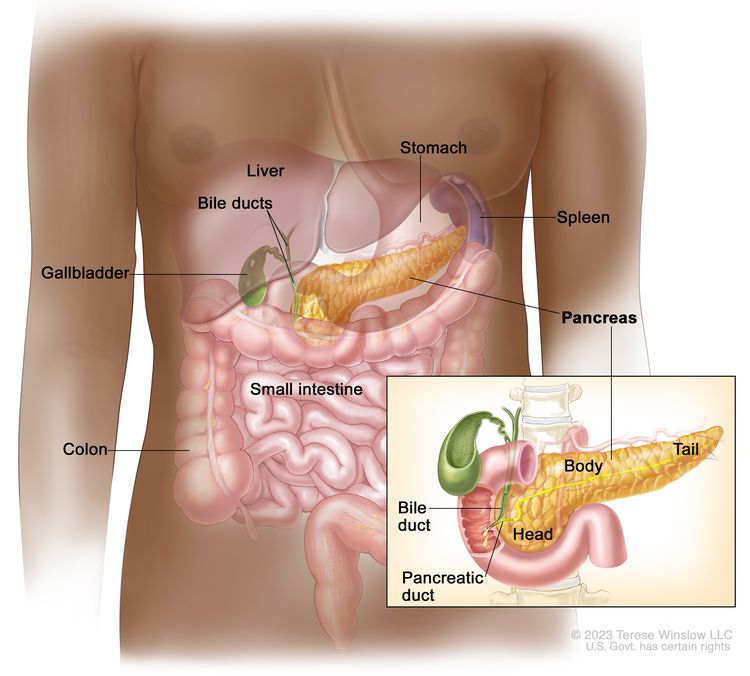This detailed medical diagram illustrates the digestive tract of a light brown-skinned male figure, from the shoulders to the pelvis area. The body is slightly faded, allowing visibility into the internal organs. Prominently labeled organs include the stomach, liver, bile ducts, gallbladder, colon, small intestine, pancreas, and spleen. The liver appears pink, the bile ducts and gallbladder are green, the stomach is pink, the spleen is purple, and the pancreas, resembling a corncob, is yellow.

In the lower right, a beige rectangle zooms in on the pancreas, displaying the tail, body, head, bile ducts, and pancreatic duct in more detail. The pancreas within this close-up is highlighted with additional colors—pale pink, green, and yellow—to stand out. The remainder of the diagram features pale pink organs, with black lines connecting them to their respective labels in black text. The image is marked with "2023 So Wenzel LLC U.S. Government has certain rights" in the bottom right corner.